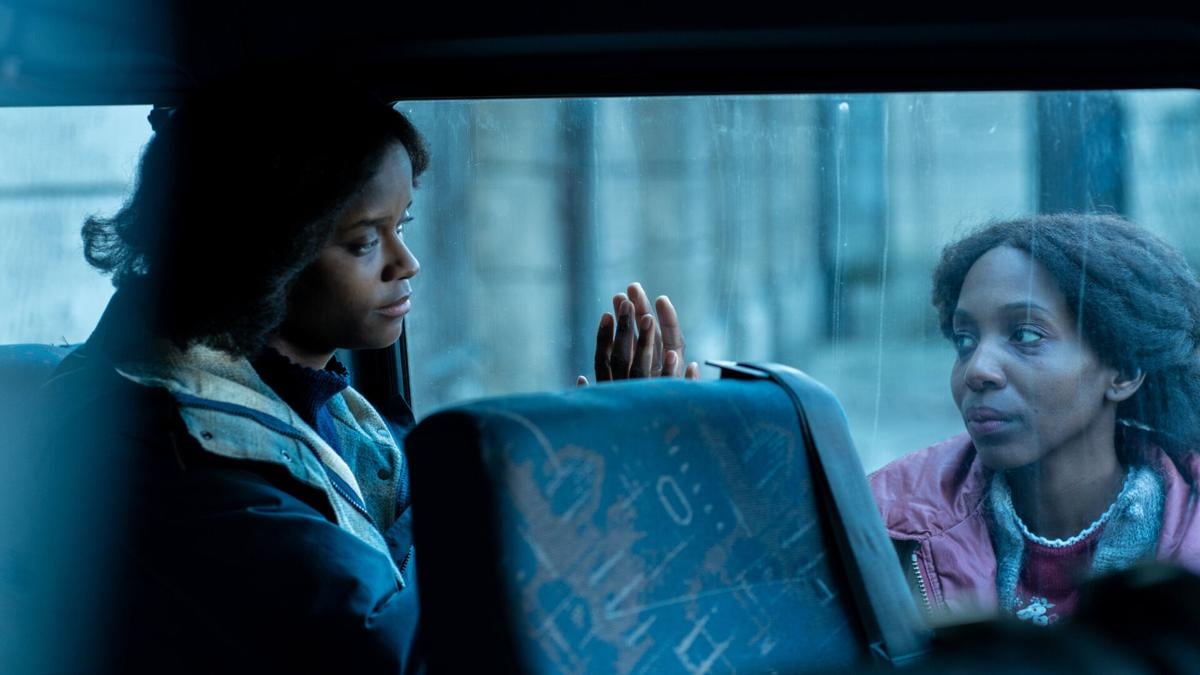In this image, two women are on opposite sides of a bus window intensely engaging with each other. The woman outside the bus, a black woman with long black hair pulled back, is seen wearing a purple jacket over a dark purple shirt with a white neckline. She has a solemn expression as she places her hand on the glass, mirroring the gesture of the woman inside. There are white streaks running down the glass between them. The woman inside the bus has partially obscured eyes behind her dark black hair, and she is donning a dark blue coat. Directly in front of her is the slightly sketched back of a blue seat with cream and orange marks, a horizontal black bar above completing the interior bus setting. Both women seem locked in a silent moment, hands pressed against the same spot on the glass, creating an evocative and emotional scene.